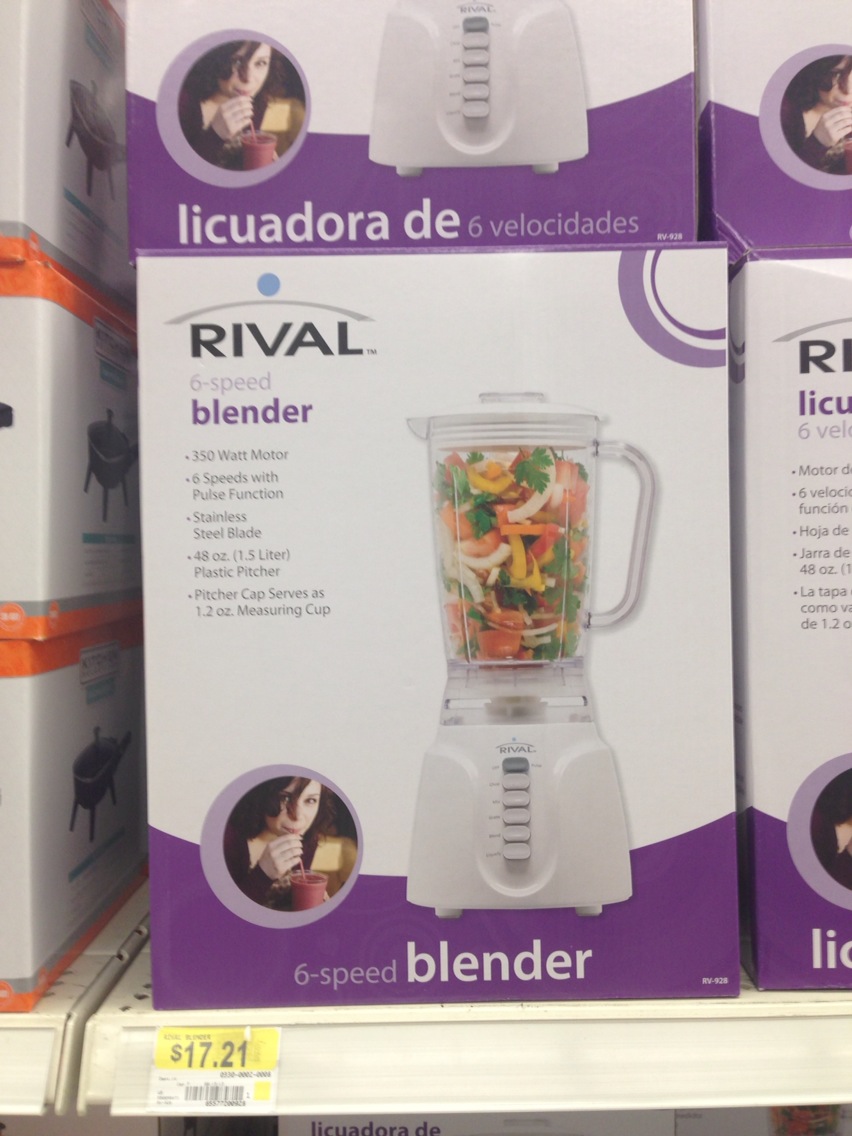This photograph captures a retail store shelf displaying several blenders, prominently featuring the Rival brand six-speed blender. The eye is drawn to the largest box at the center, which shares the shelf with identical models. The blender is white with a transparent 48-ounce (1.5-liter) plastic pitcher, highlighted on the box by a photograph of the blender filled with various vegetables. The product’s key features listed on the box include a 350-watt motor, stainless steel blades, pulse functions, and a pitcher cap that doubles as a 1.2-ounce measuring cup. The packaging design is mainly white with a distinctive purple border. Additionally, there’s a smaller image of a woman drinking a smoothie made with the blender. The yellow price tag shows it is priced at $17.21. The shelf also holds other items, including a white box with orange and gray accents that appear to be a grill or another cooking appliance. The shelf itself is white, contrasted by its metal structure.